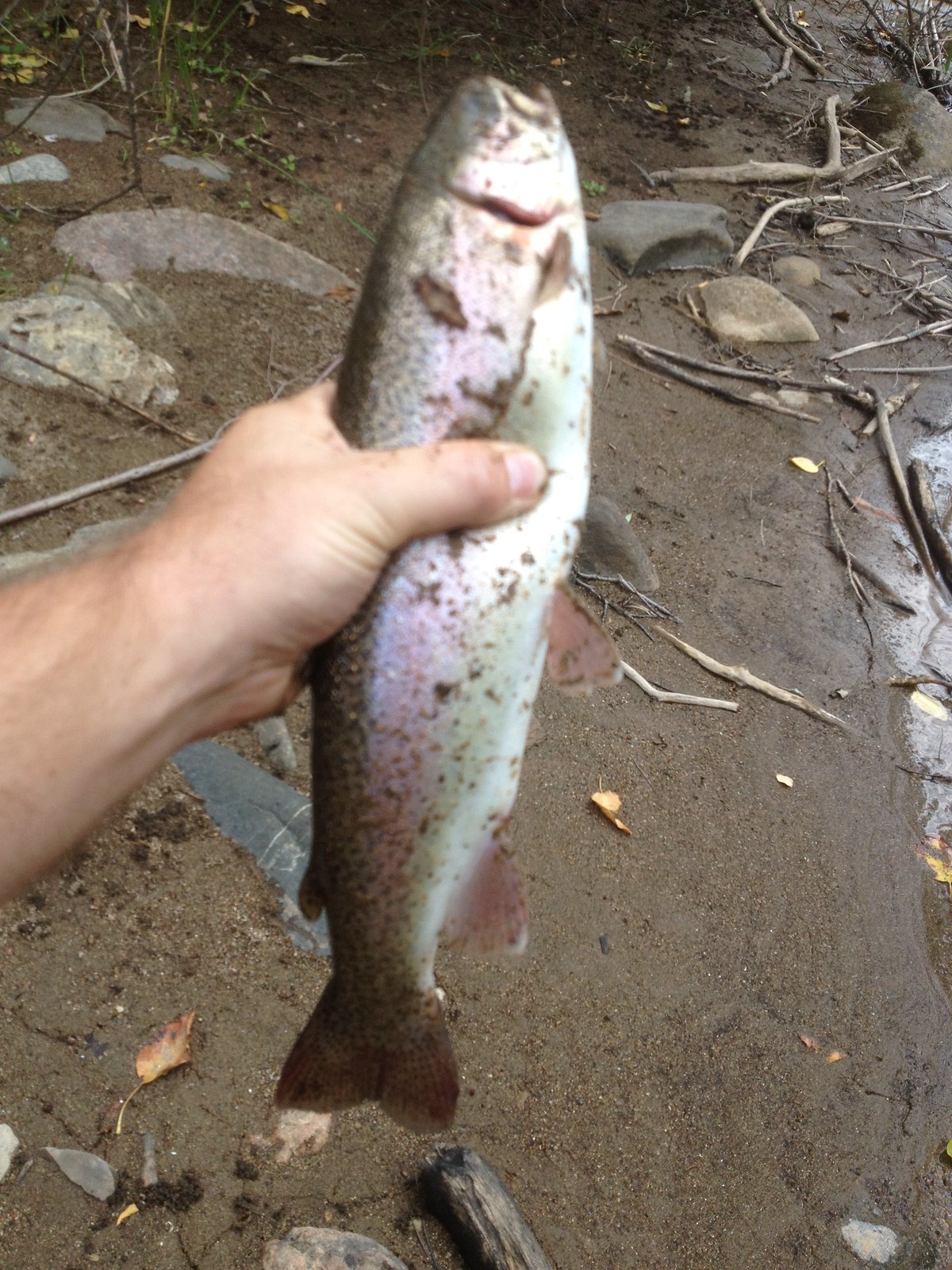The photograph is a vertically aligned color image taken outdoors on a cloudy day, at the muddy edge of a lake or river. It prominently features the left hand and part of the arm of an adult Caucasian man, holding a freshly caught rainbow trout. The fish, displayed head up and tail down, showcases a beautiful array of speckled purples and silvers along its length, measuring approximately 12 to 14 inches. The scene around the fish is distinctly wet and muddy, littered with rocks, sticks, driftwood, and scattered leaves. The man's hand emerges from the left middle portion of the image, firmly grasping the fish, emphasizing his catch against a backdrop that includes wet sand, half-buried stones, and branches from a nearby bush or tree.